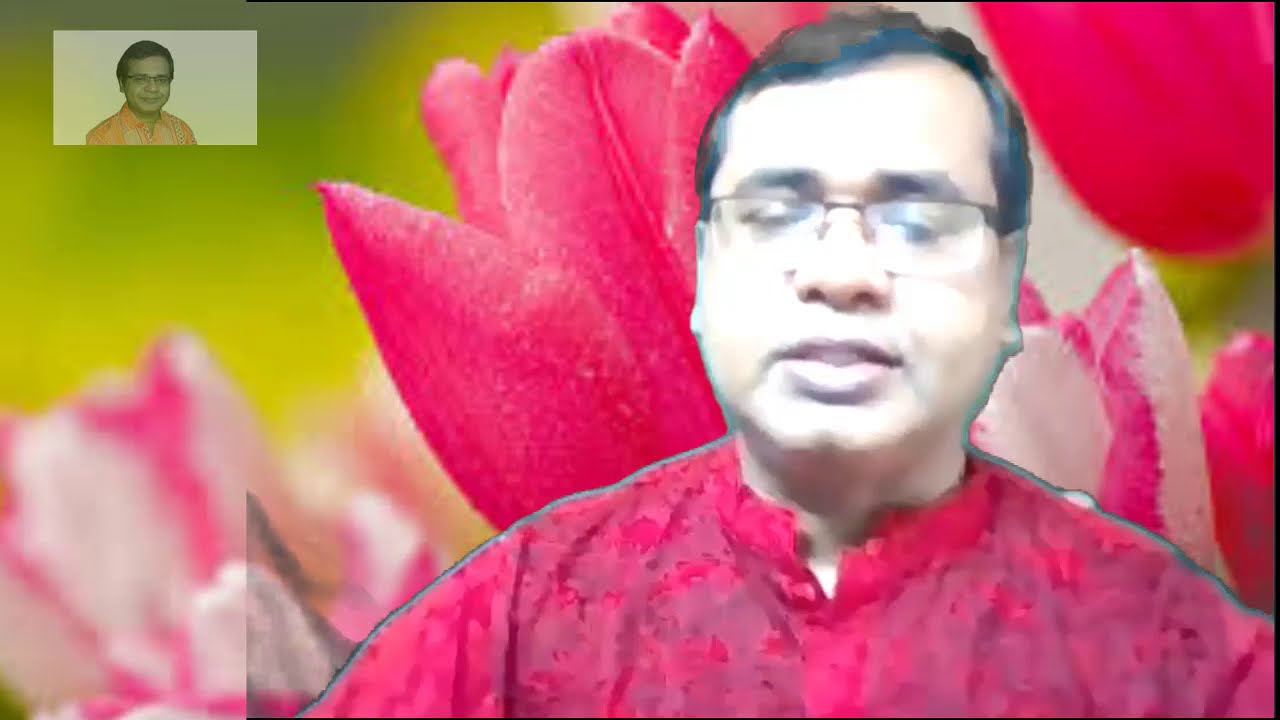The image depicts an Indian or Pakistani man with tan skin, short black hair, and glasses. He appears to be on a video call or videoconference, as evident from his red shirt with a tall collar. His eyes seem heavily closed. The background is digitally enhanced, resembling a green screen. This artificial backdrop features a collection of large red and white flowers with intricate red patterns. In the farthest part of the background, there are various hues, primarily green and orange, and green and yellow colors. Located at the top left corner is a small red rectangle containing another picture of the same man, this time wearing a yellow or orange shirt. This composite image appears to be a screenshot from a platform like Zoom, devoid of any text, and the primary subject is positioned towards the right side of the frame. Various colors including pink, purple, brown, black, white, and silver are visible.